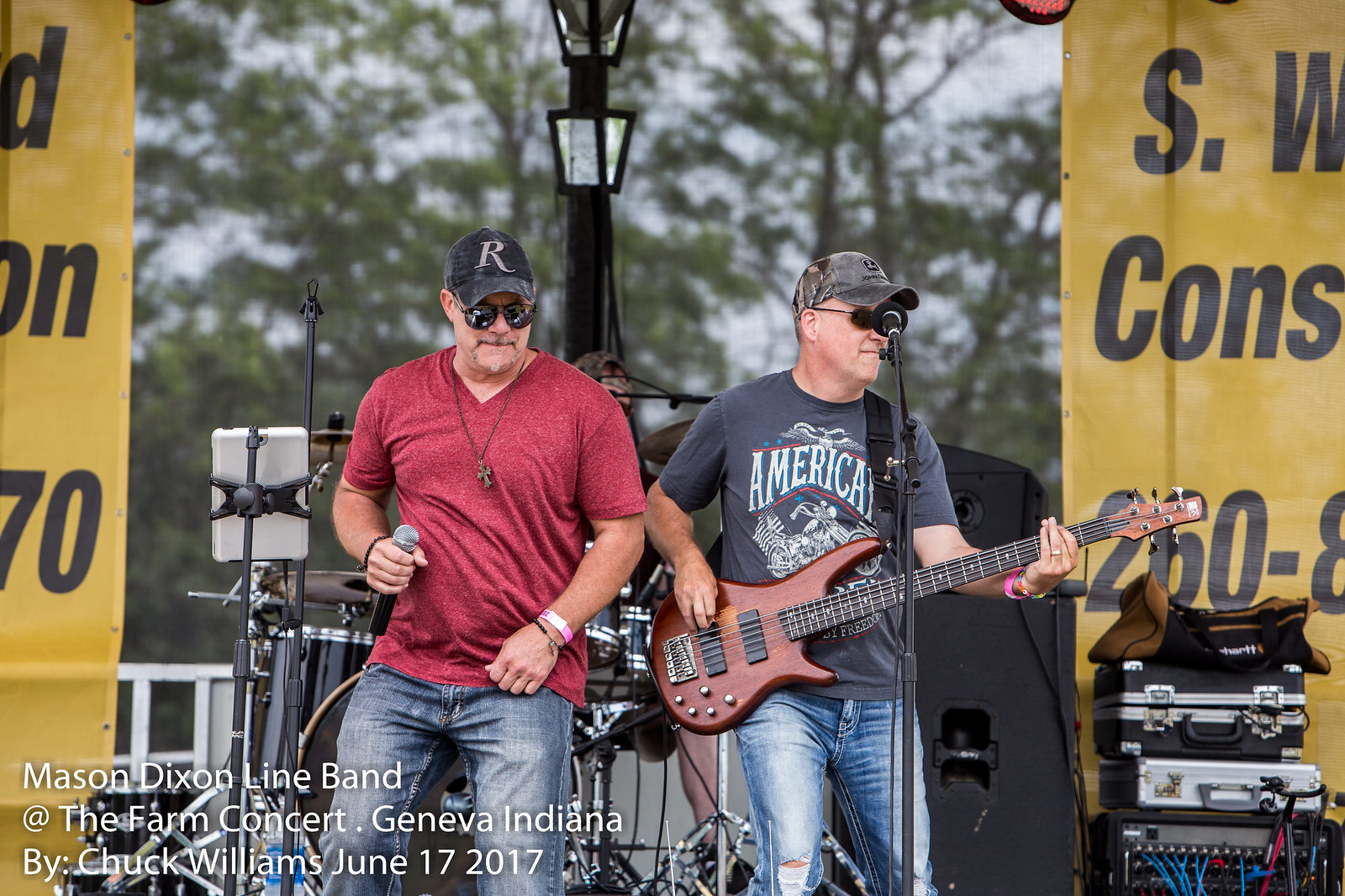This photograph, taken by Chuck Williams on June 17th, 2017, captures the Mason-Dixon Leather Band performing a concert in Geneva, Indiana. The stage is set outdoors, framed by a backdrop of trees and a lamppost. Two male band members are seen in the foreground, each wearing black hats, sunglasses, and blue jeans. One is dressed in a black T-shirt emblazoned with the word "America" and holds a dark wood-colored electric bass. The other wears a red T-shirt and is captured holding a microphone, fully immersed in the performance. Behind them, musical equipment, speakers, and microphones clutter the stage. Two large yellow banners with black lettering—though partially obscured—hint at the event's sponsors. The overall vibe is vibrant and dynamic, as the band jams energetically before their audience.